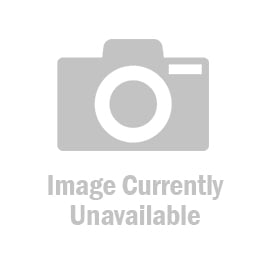On a white background, there is a vintage Statico model number 52010 surface resistance checker, designed to measure ohms per square. The device itself is flat and constructed from black or possibly brown plastic or Bakelite. It features a prominent yellow rectangular inlay on the front, where the details and readouts are displayed. The inlay contains text indicating various resistance levels, ranging from 10^3 (conductive) to 10^12 ohms per square (insulative), with intermediate values labeled as static dissipative. Positioned centrally on the inlay is a red button labeled "test." To the right of this button is a hole labeled "ground," intended for grounding purposes. Accompanying the checker is the probe and cable, which connect to the main device, allowing it to function as a measuring instrument.